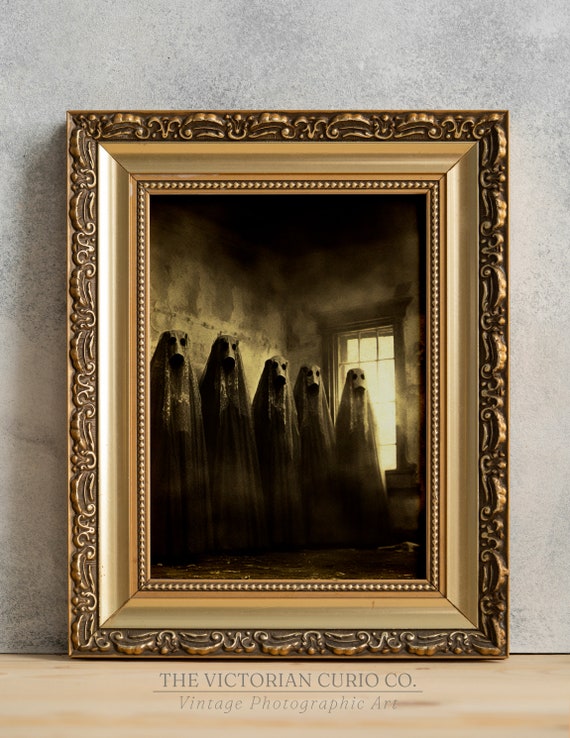The image features an ornate, rectangular golden picture frame with detailed accents and wavy textures, leaning against a gray wall and resting on pine-colored flooring. Inside the frame is a black and white photograph labeled "The Victorian Curio Co. Vintage Photographic Art." The photograph depicts five hooded figures, resembling classic sheet-overhead ghosts, standing in a line within a barren, unpainted room. The hooded figures have eye and mouth holes cut out, suggesting masked faces, and wear dark, robe-like garments. One figure stands in front of a barred window, through which bright sunlight streams, highlighting the eerie and potentially cursed nature of the scene. The overall atmosphere is spooky and unsettling, fitting of the vintage, haunted aesthetic implied by the label.